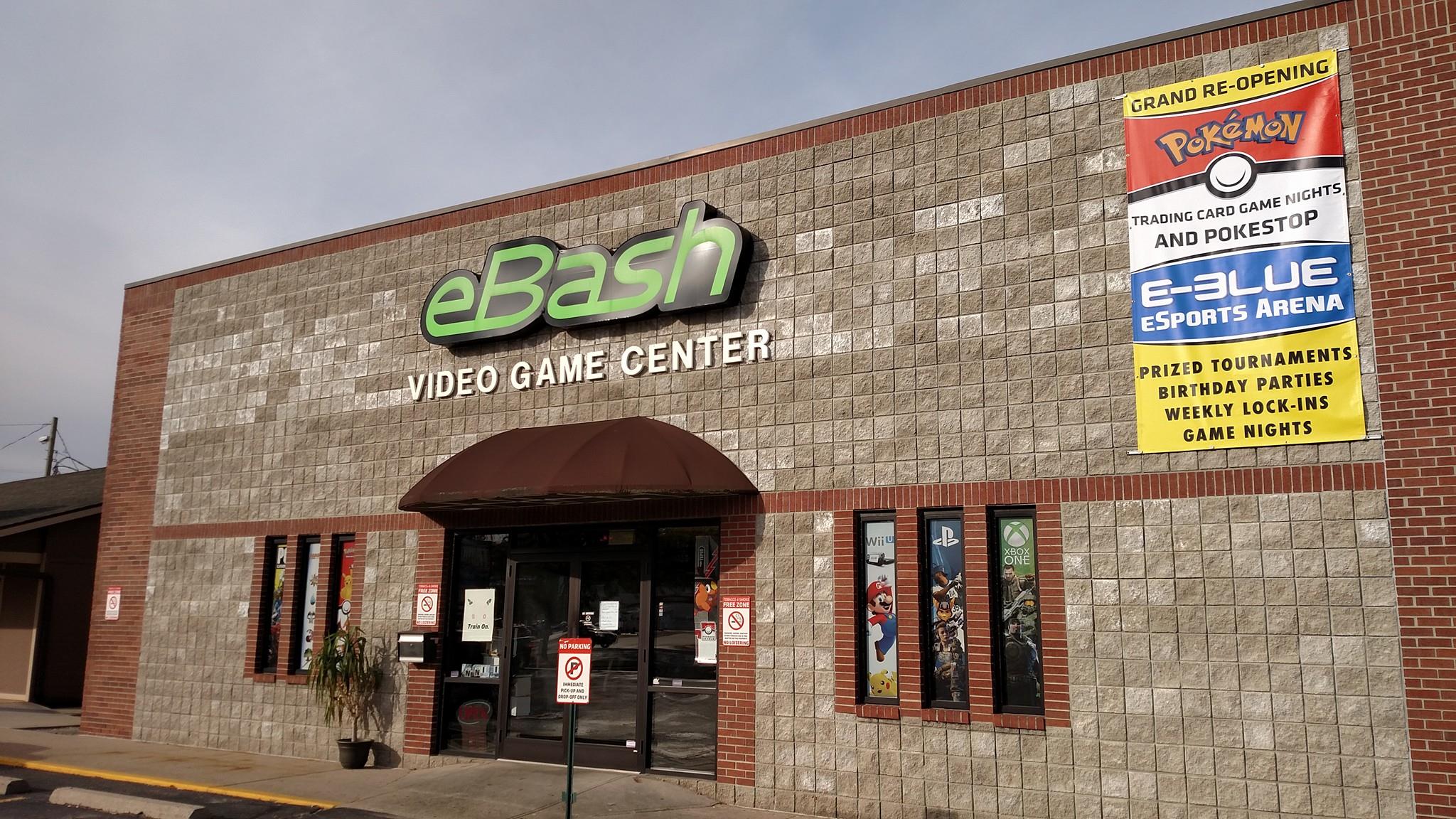In the foreground of this horizontally oriented photo, you see the front of the eBash Video Game Center, a large two-story brick building. The facade features a mix of gray concrete tiles and traditional red bricks, giving it a robust and industrial aesthetic. Centered above the entrance, the eBash logo is prominently displayed in vibrant green and black. Below, there are glass double doors flanked by narrow windows, creating a welcoming entryway beneath a protective red or brown awning. The doors bear essential signs, including a no parking notice that designates the area for pick-up and drop-off only.

To the left, glimpses of an adjacent building are visible, and power lines stretch across the background, adding to the urban atmosphere. In the upper-right corner of the building, a banner hangs, heralding a Grand Reopening and advertising various community activities such as Pokemon Trading Card Game Nights, eBlue Esports Arena events, prize tournaments, birthday parties, weekly lock-ins, and game nights. This banner underscores the building's role as an active, family-friendly hub for gamers of all ages.